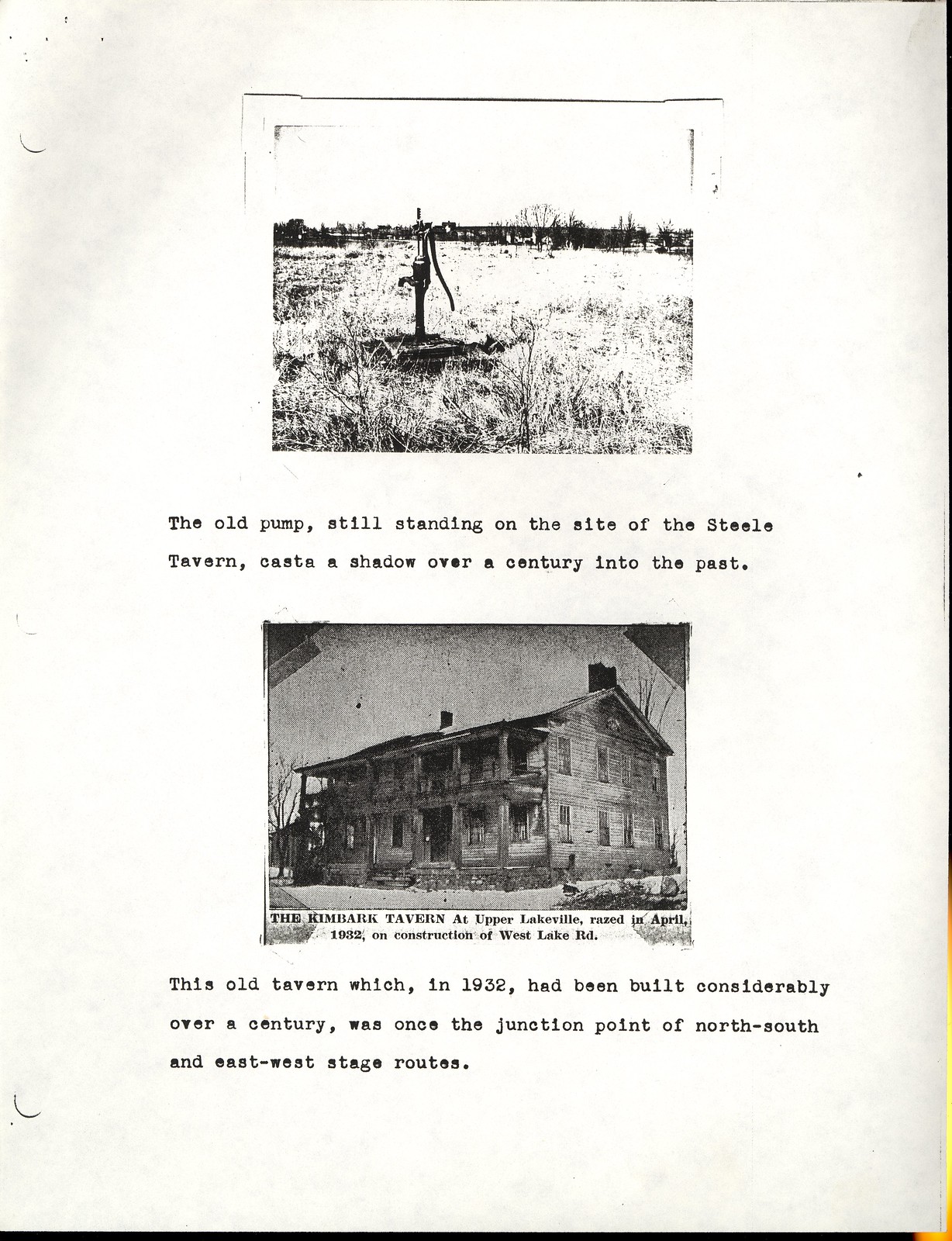This detailed black-and-white scan of a slightly off-white, slightly folded sheet of paper, likely part of a larger document, features two historic photographs and typewritten text. The paper shows signs of being photocopied, including punched holes for a three-ring binder.

The top photograph depicts an old-style upright water pump in a barren field of what appears to be dead grass. In the background, faint silhouettes of trees and possibly buildings can be discerned. The overlaying text reads, "The old pump, still standing on the site of the Steel Tavern, casts a shadow over a century into the past."

The second image showcases a large, wood-framed, two-story house set at an angle, with a peaked roof and chimneys at both ends. The house, adorned with numerous windows – at least five on each floor on the front and three on each side – also features a prominent porch. The accompanying text notes, "The Kimbark Tavern at Upper Lakeville raised in April 1932 on the construction of West Lake Road. This old tavern, considerably over a century old by 1932, once served as the junction point for North-South and East-West stage routes."